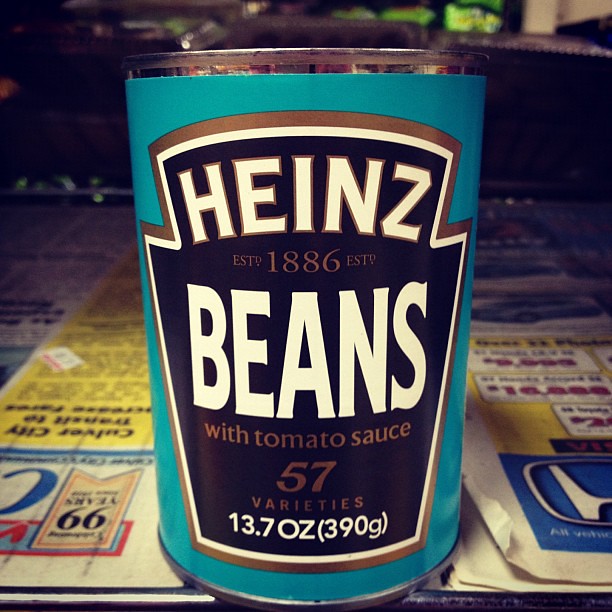This square, indoor digital photograph centers prominently on a can of Heinz beans in tomato sauce. The tin can, featuring a vibrant blue label, dominates the frame against what appears to be a magazine or newspaper backdrop showcasing car advertisements from a Honda dealership. The upper part of the image reveals a darker brown or black surface, possibly a countertop.

The Heinz beans label is distinguished by a crest-shaped logo in black with a white and gold outline. In white text, it reads "Heinz beans," and in gold, "EST. 1886." Below this, it states "with tomato sauce" and "57 varieties" in gold lettering. At the bottom of the label, "13.7 OZ" and "(390 G)" are noted in white font. Silver accents, including the can's top, add a metallic contrast to the scene.

Surrounding the can, the newspaper/magazine features vivid elements: a blue square with the Honda logo, yellow advertisements detailing car deals with white boxes and red pricing, the phrase "99 years" upside down on a bookmark-like section on the left, and a prominent yellow column with black text. These details frame the can, hinting at its placement on a casually set table laden with printed materials.